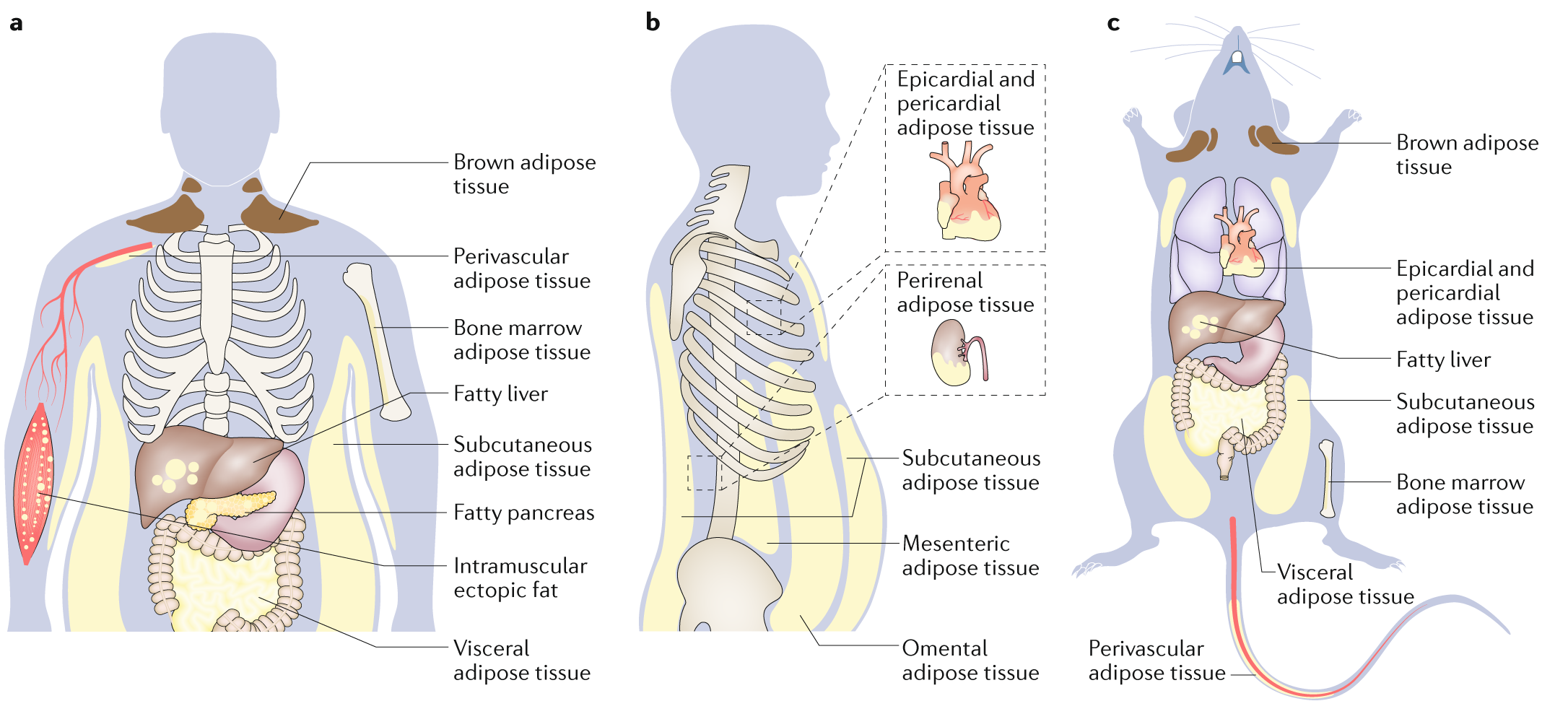The image is a horizontally oriented informational graphic divided into three panes labeled A, B, and C. Each pane features a detailed outline of anatomical structures for comparison and educational purposes. Pane A presents a front view of a translucent human silhouette labeled with black text pointing to different types of adipose tissue—such as brown adipose tissue, perivascular adipose tissue, subcutaneous adipose tissue, and visceral adipose tissue—as well as specific internal organs like the liver and pancreas, indicating conditions like fatty liver and fatty pancreas. Pane B shows a side view of the same human figure, depicting additional anatomical details including the bones (sternum, ribs, vertebrae), the liver, heart, and varied adipose tissues like epicardial, pericardial, and perineal adipose tissue. Beside Pane B are breakout boxes illustrating a heart and kidney. Pane C contrasts these details with a similar outline of a rat, highlighting analogous internal organs such as the lungs, heart, liver, and intestines, along with labels for subcutaneous and visceral adipose tissue. This comparative graphic appears to be a medical or biological training document, emphasizing the similarities and differences in adipose tissue distribution and internal organ structures between humans and rats, possibly in the context of studying metabolic diseases.